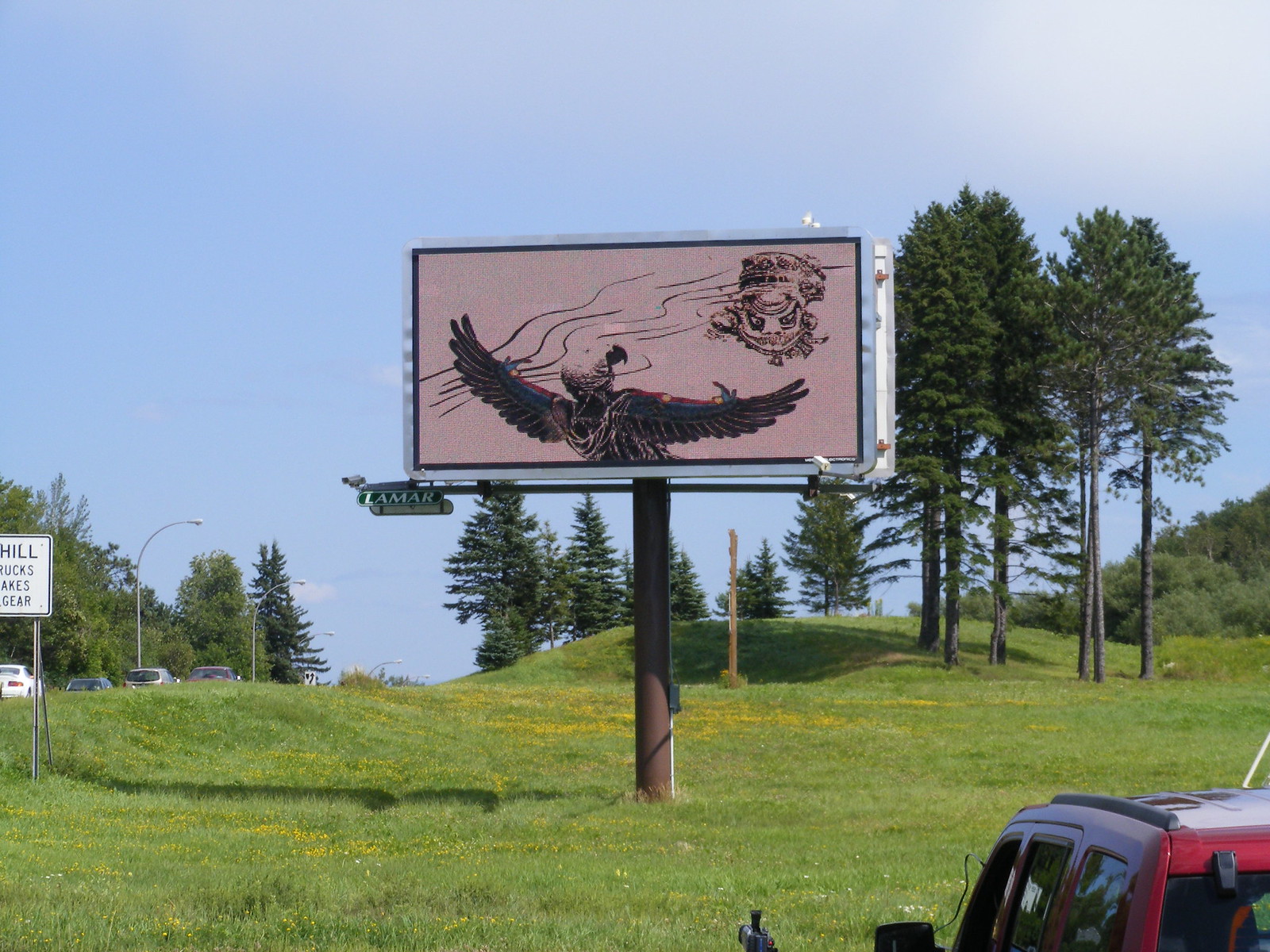This photograph captures a white billboard with black trim, standing prominently in the center of a lush, green, park-like area. The billboard is held aloft by a thick wooden pole that casts a shadow on the grassy ground below, dotted with patches of yellow dandelions. The primary image on the billboard is a large eagle, wings spread wide, sketched in black and white, dominating the bottom center. In the upper right corner of the billboard, there is a character with a face that resembles the Mad Hatter from "Alice in Wonderland" wearing a hat. To the left, partially peeking out from behind the main sign, another sign reads "Hill, Trucks, Axes, Gear" in black lettering. The scene is framed by evergreen trees, bare along their trunks with full foliage at the top, and a distant mountainous area, adding a serene backdrop. A red car is parked to the right of the billboard, and several other cars are lined up facing away from the camera.